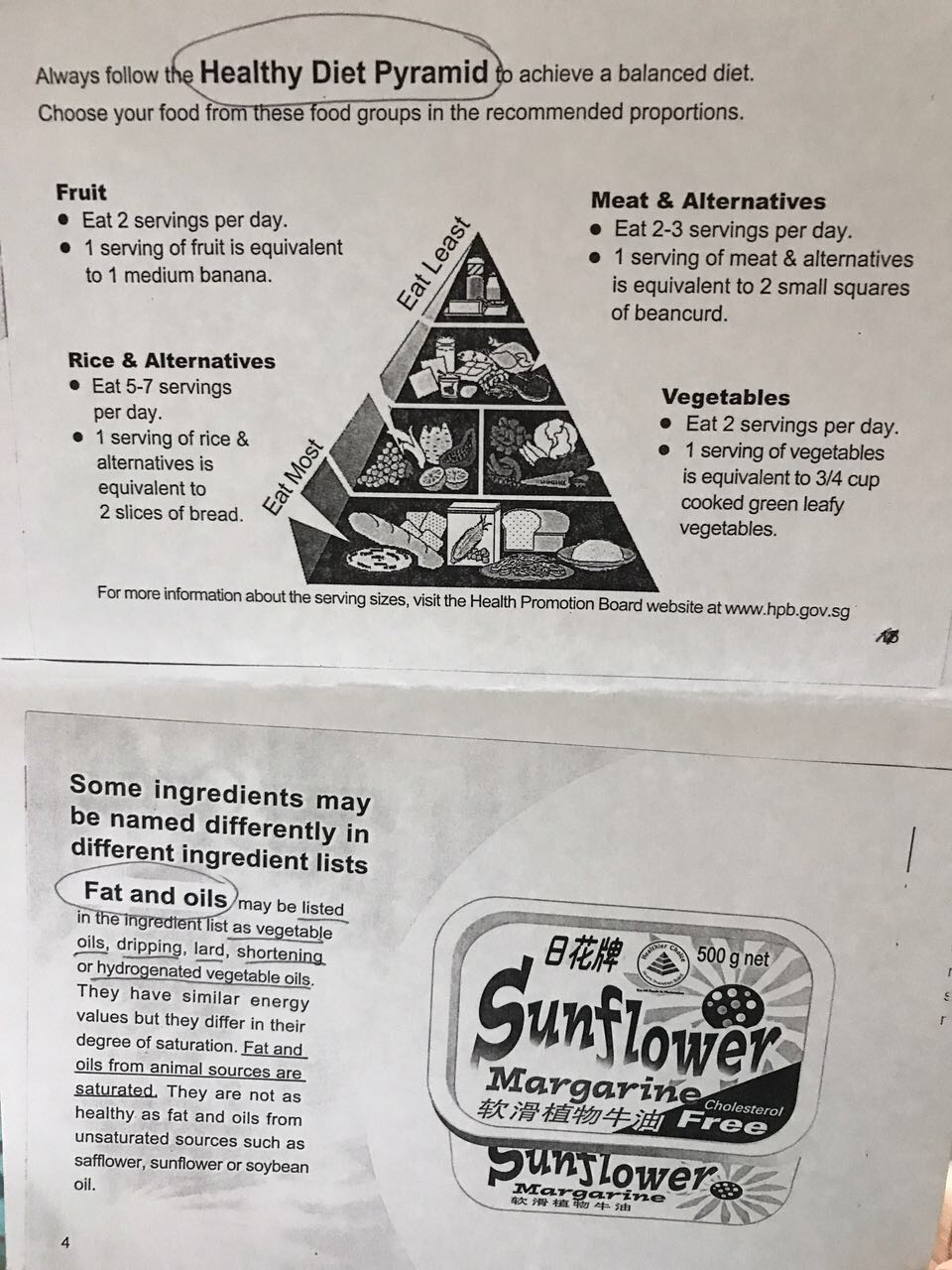This photograph captures a detailed flyer and an additional informative paper, both predominantly in black and white text, set against a white background. The top flyer is titled, "Always Follow the Healthy Diet Pyramid to Achieve a Balanced Diet. Choose Your Food from These Food Groups in the Recommended Proportions." The phrase "Healthy Diet Pyramid" is circled with a pen. The flyer is divided into four sections: Fruit, Rice and Alternatives, Meat and Alternatives, and Vegetables. Each section contains advice on recommended servings: Fruits (2 servings), Rice and Alternatives (5-7 servings), Meat and Alternatives (2-3 servings), and Vegetables (2-3 servings).

Centrally featured on the flyer is a food pyramid, segmented to show the different food groups. The pyramid starts with "Eat Most" at the bottom, encompassing broad categories such as bread, followed by fruits and vegetables, then meat and alternatives, and finally, "Eat Least" at the top, for items like processed sugars.

The bottom of the page guides readers to visit the Health Promotion Board website (www.hpb.gov.sg) for more information on serving sizes.

Beneath this flyer is another piece of paper discussing ingredient labeling, specifically fats and oils. It notes that some ingredients might be named differently in various ingredient lists. This page elaborates on fats and oils, highlighting hydrogenated vegetable oils, and mentions that fats from animal sources are typically saturated and less healthy compared to unsaturated fats from sources like sunflower or soybean oil. The term "Fats and Oils" is circled, and various phrases such as "vegetable oils," "drippings, lard," "shortening or hydrogenated vegetable oils," and "saturated fats from animal sources" are underlined for emphasis.

To the right of this explanatory text, there's an illustration of a tub of sunflower margarine labeled "Cholesterol Free" with a sun icon and some Chinese characters, providing a visual reference to healthy unsaturated fat choices.